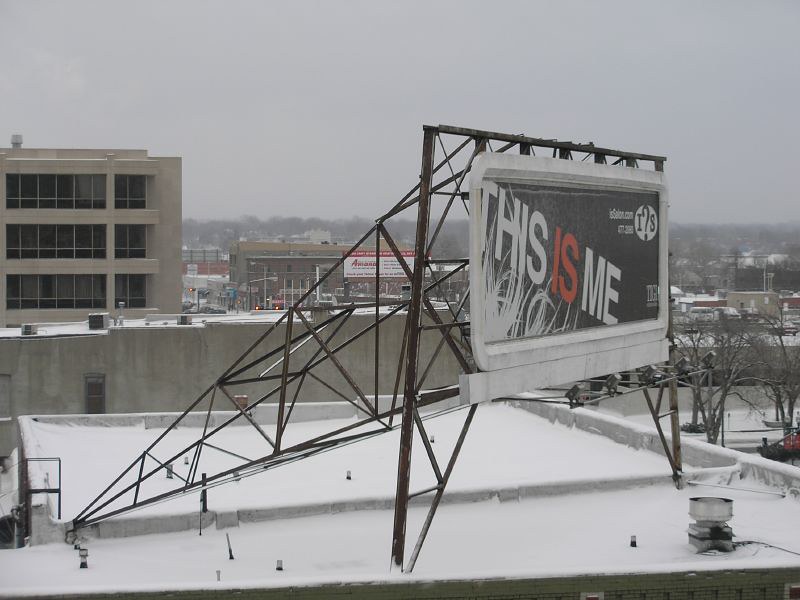The image depicts a slightly wider-than-tall color photograph of a snow-covered, flat business rooftop. Prominently featured in the lower right-hand corner is a commercial air intake. The rooftop hosts a billboard, held up by dark grey, crisscrossing scaffolding positioned roughly in the direction of four to five o'clock. The billboard has a thick white border framing a black background, with the text "This is me" sprawled across it. The words "This" and "me" are presented in white capital letters, while "is" is in a medium red color. Below the text, white grass-shaded lines are included, adding artistic flair to the billboard. In the upper right corner of the billboard, there is a mysterious white circle with indistinct black markings. Behind the rooftop, a grey, three-story building with a cement base is partially visible. Additionally, another building in the background features red and white signage. The overall scene is set against a grey, cloudy sky with distant, colorless trees adding depth to the horizon.